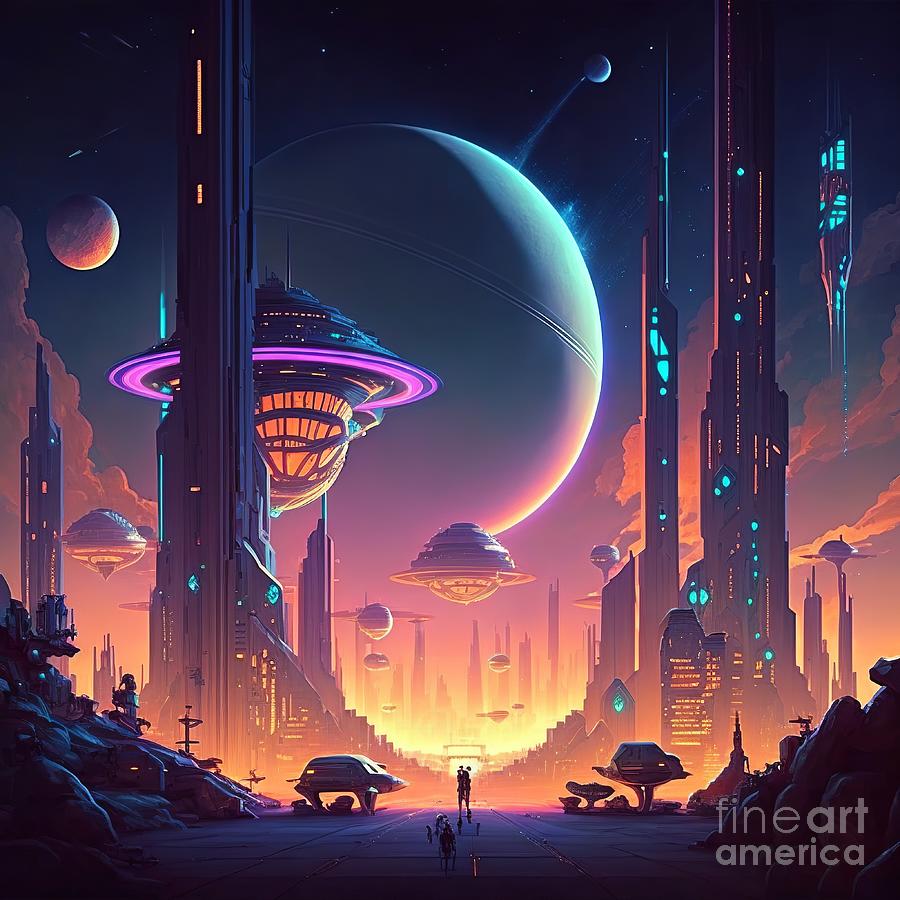This vibrant, square, full-color artwork captures a vivid sci-fi scene, with no borders and a watermark labeled 'Fine Art America' in the lower right-hand corner. The foreground showcases a street where two people stand, surrounded by rugged rocks and lush trees. To their left, there's a futuristic vehicle, while the right side features another vehicle on a distant stand. Beyond them, the scene transitions into an urban landscape, teeming with towering skyscrapers, some of which extend beyond the frame, merging into the vibrant sky. 

This skyline is dotted with floating satellite devices and various structural elements that add to the futuristic ambiance. The backdrop is a blue sky adorned with sporadic white stars, adding to the outer space theme. Dominating the upper left and upper right are two prominent moons, accompanied by a vast planet that looms in close proximity, adding scale and depth to the scene. The sky bursts with shades of blue, purple, yellow, and orange, imparting an almost animated, CGI-like quality to the art piece.

Overall, the image is a feast of color and detail, strikingly merging natural and extraterrestrial elements to portray a vivid, otherworldly urban spectacle.